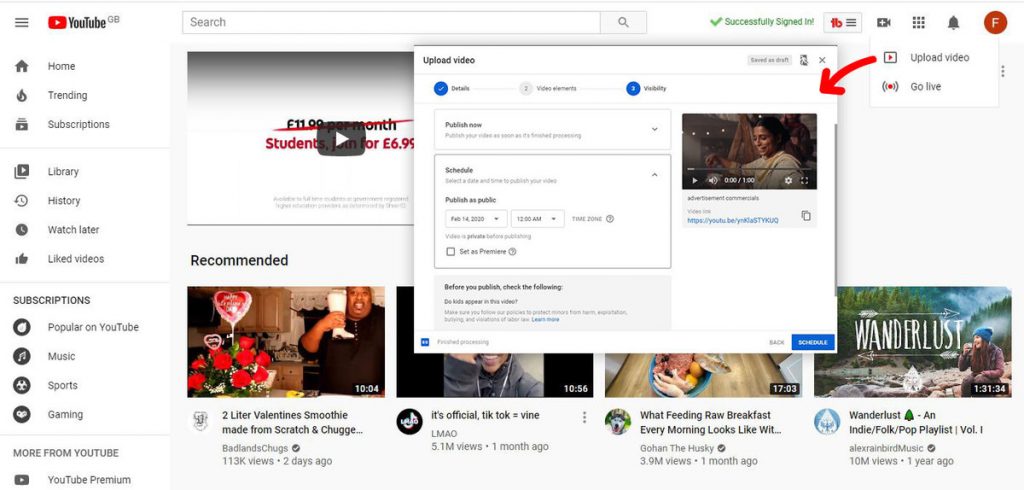A screenshot from a YouTube page shows a pop-up box with the title "Upload Video" at the top. Below this header, the interface is divided into three clickable sections: "Details," "Video elements" marked with a number '2,' and "Visibility" marked with a number '3'. There is a hand-drawn red arrow on the left side of the screen pointing from a smaller dropdown box situated in the upper right corner that contains buttons for "Upload video," denoted with a play icon, and "Go live," signified by a signal icon. The arrow targets the main "Upload Video" box.

Within the upload interface, there's an advertisement commercial video being uploaded. The user has scheduled the video for publication on February 14th, 2020, at 12 a.m., as specified in the scheduling boxes. The pop-up also includes a section labeled "Before you publish, check the following," which prompts the user to confirm if kids appear in the video. More information about this query is available for further reading.